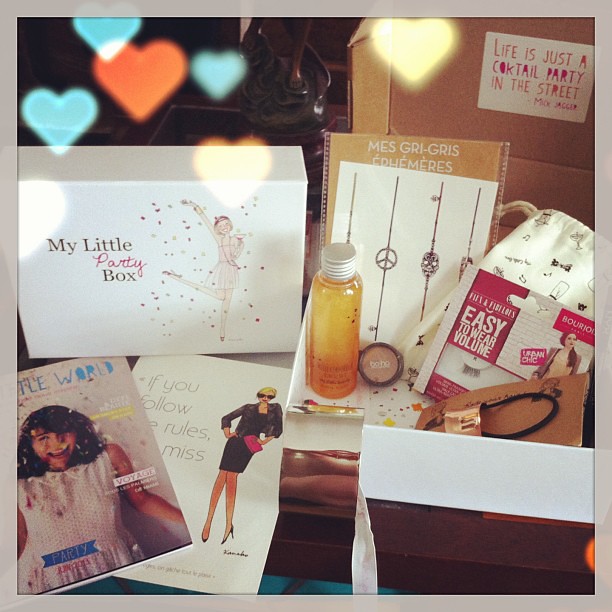A vertical rectangular image displays an intricately arranged collection of items, reminiscent of a curated display at a vendor's booth or a celebratory gift box arrangement. The background features a narrow white border surrounding the image, adorned with small superimposed hearts in the upper right and lower left corners. The setting suggests a cozy indoor environment, with a possible wall on the right side and a window on the left, through which stars can be faintly seen along with some hanging hearts.

At the center of the composition sits a prominent white box labeled "My Little Party Box," featuring a festive illustration of a woman surrounded by confetti. The box appears to be the focal point of the display. Surrounding the box, there is an assortment of items spread across what appears to be a coffee table. To the right of the box, beauty products and jewelry occupy distinct compartments, including a black-and-white fabric gift bag and a small drink container or bottle.

In the lower right corner, there are magazines with partially visible covers—the one most noticeable features a smiling girl in a white dress amid falling confetti, while another adjacent magazine features a stylish, cartoon woman and text that reads "If you follow the rules," partially obscured by the first. Additionally, there are various trinkets including fake eyelashes, stickers, a hair clip or hairband, and possible greeting cards or notebooks scattered around. 

Overall, the meticulously arranged objects, varying from beauty products to celebratory paraphernalia, evoke the sense of a thoughtfully prepared gift ensemble, captured in a photograph to showcase the curated collection.